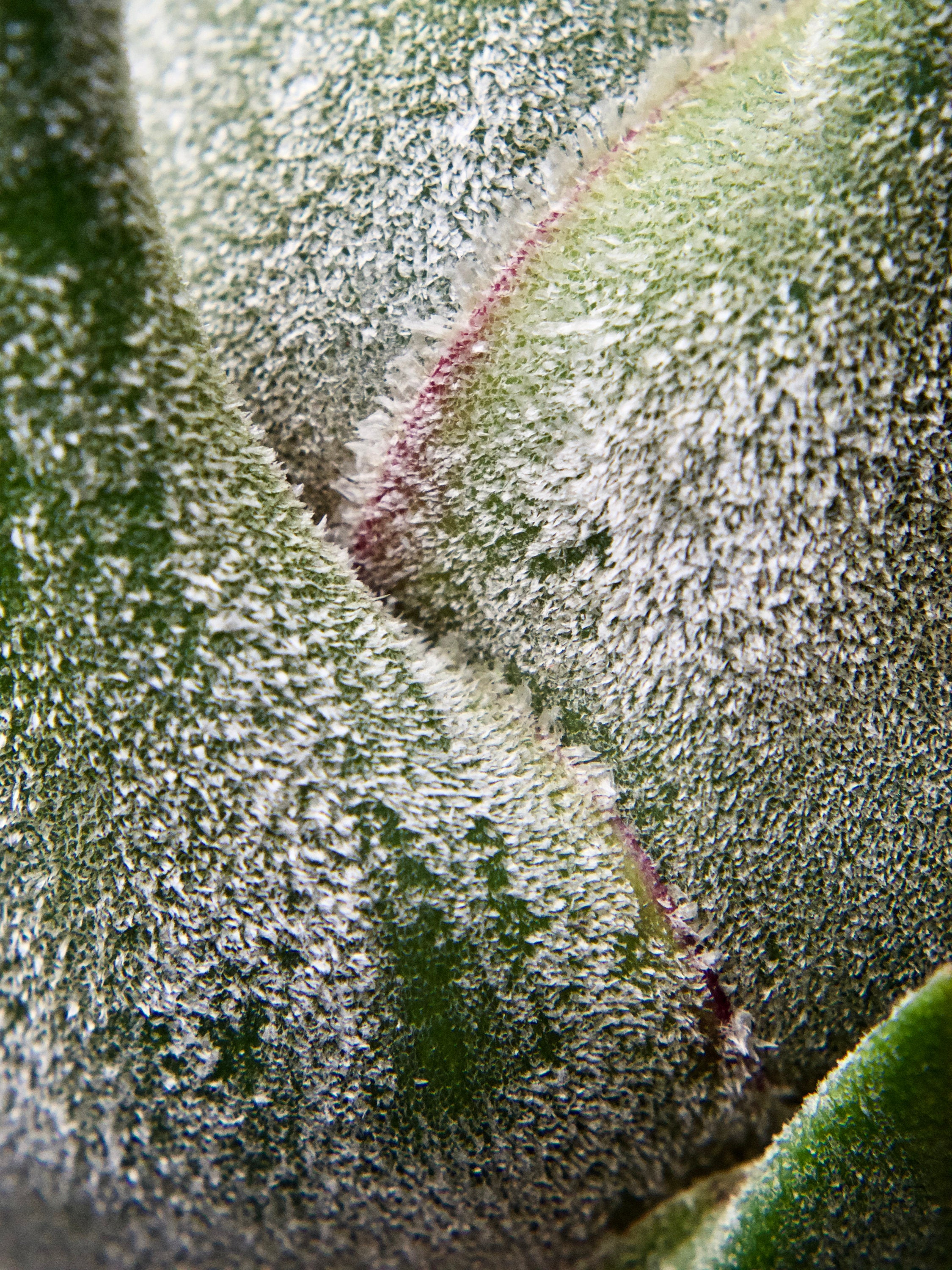This intriguing and detailed close-up image appears to depict a leaf adorned with a layer of frost or snow. The photograph, which is highly magnified, showcases the leaf's vibrant green hues, ranging from dark green to medium green, with intricate lighter green patterns. A prominent red line starts from the top left, curving downward, flanked by a yellowish line on one side and a pink line on the other, forming a V-shape that extends towards the top right corner. The surface of the leaf incorporates another red line descending near the right, accentuating its curvy structure. The entire scene is encrusted with white, flaky crystals, giving it a frozen, fuzzy appearance. The overlay of frost and snow on the leaf's textured surface presents a captivating contrast, blending the natural vibrancy of the leaf with the stark, crystalline beauty of a wintry coat.